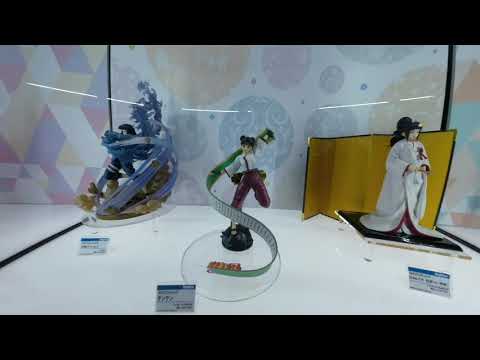The image captures a color photograph of three intricate Asian art figurines displayed within a glass case, reflecting light and possibly the silhouette of the photographer. The figurines are placed against a subtle white background adorned with light-colored decorations and accompanied by small descriptive tags featuring a blue stripe on top. 

To the right, a detailed figurine of an Asian woman with black hair stands resplendent in a long, elaborate white robe accentuated with a red ribbon, positioned in front of a gold and black folding screen. In the center, another figurine portrays a girl with black hair, dressed in a white top and red pants, with a large, green and white strap artistically flowing around her. To the left, a blue sculpture, possibly representing a dragon-like form, adds a contrasting hue to the display. The scene is further enhanced by orbs and circles of various colors—red, orange, green, and blue—in the background, lending a vivid and dynamic atmosphere to the display.